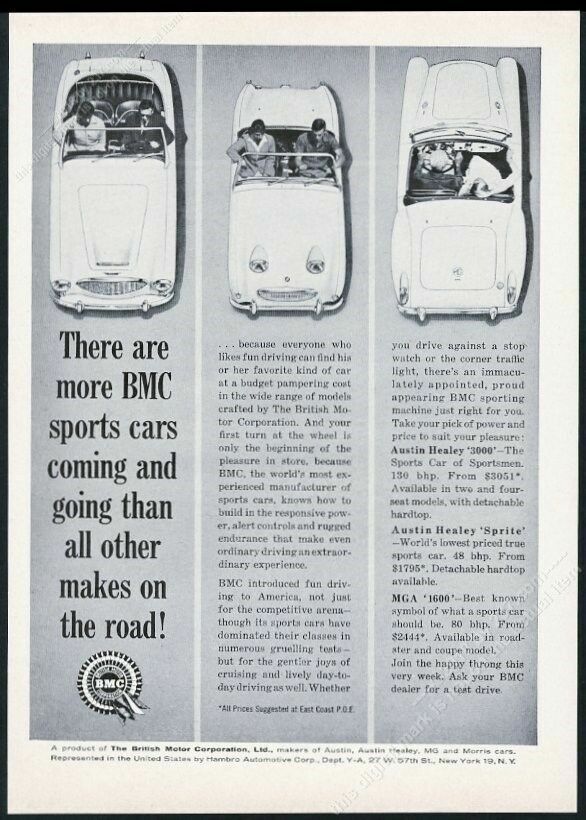This detailed caption can help clearly describe the image based on the gathered information:

The image depicts a vintage black-and-white newspaper or magazine advertisement, framed in black with a beige matting. The ad promotes the British Motor Corporation (BMC) and prominently features the bold text: "There are more BMC sports cars coming and going than all other makes on the road." At the top of the image, three different BMC car models, likely set in white due to the monochromatic nature of the photo, are displayed side by side. The models are identified as the Austin-Healey Sprite, MGA 1600, and the Austin-Healey 3000. The cars, each with visible passengers, represent a long vehicle with a passenger seat placed far back, a smaller compact vehicle, and a roadster-style car respectively. Below the main text is the BMC logo and the statement "A product of the British Motor Corporation, LTD." The article elaborates on how BMC has introduced fun driving cars to America, appealing not just to competitive drivers but to anyone with a love for driving, stressing affordability and variety in their offerings. Additionally, pricing details, such as the Austin-Healey 3000 starting at $3,051, are highlighted on the right side of the ad.